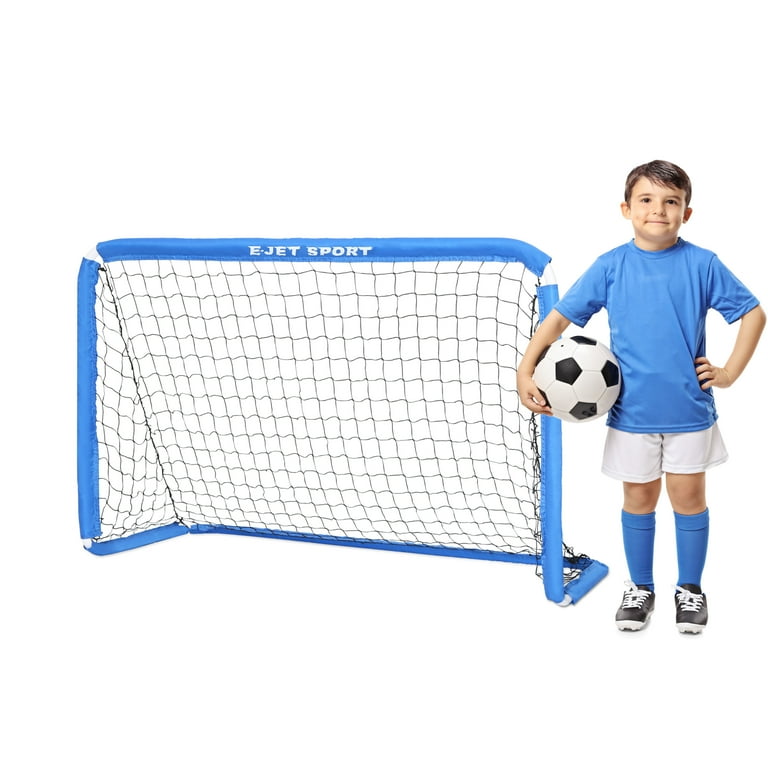The photograph features a little boy, estimated to be between 8 and 10 years old, standing next to a soccer goal. The goal, emblazoned with "E JET SPORT" in white letters on its light blue frame that matches the boy's shirt and knee-high socks, stands at about his shoulder height. The boy is grinning and has side-swept brown hair. He wears a light blue t-shirt, white shorts, and black soccer cleats with white laces and soles. His left hand rests on his hip while his right hand holds a black and white soccer ball against his hip. The net of the soccer goal appears black, with the white background showing through the mesh. The overall scene captures a youthful, joyful moment on the soccer field.